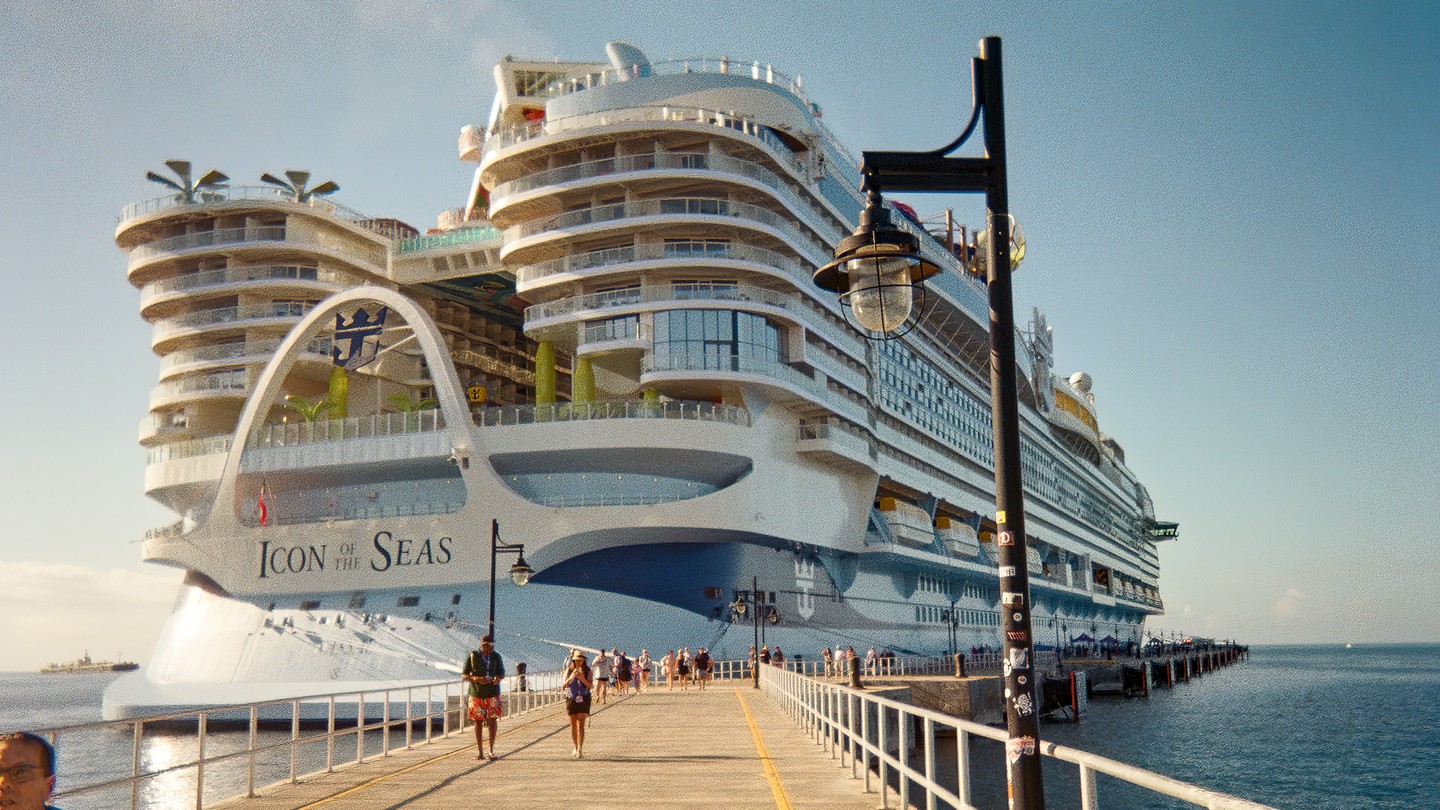The image depicts a recently built mega cruise ship, identified as the Royal Caribbean's "Icon of the Seas," docked at a pier. Taken from the pier perspective, the photograph highlights the massive vessel, towering at about eight to ten stories high, with its lower part painted in shades of blue and the upper decks predominantly white. The ship's name, "Icon of the Seas," is prominently displayed in dark blue lettering on the back, just below a distinctive white arch. 

The scene is set outdoors on a clear day, with the background featuring a blue sky transitioning to a white cloud line. The blue ocean surrounds the ship on both sides, contributing to the picturesque setting. Adding to the ship's grandeur, one of the main decks appears to have trees or greenery onboard. The ship's outboard-facing rooms are equipped with glass windows, enhancing the luxurious feel.

In the foreground, several people are seen disembarking the ship, walking along a pier-like roadway that leads away from the cruise ship. The pier is paved and lined with white fencing on both sides. Additionally, an old-time style lantern hanging from a pole is visible at the front right of the image, adding a quaint touch to the modern scene. The overall composition beautifully captures the size and elegance of the Icon of the Seas against the serene backdrop of the sky and ocean.